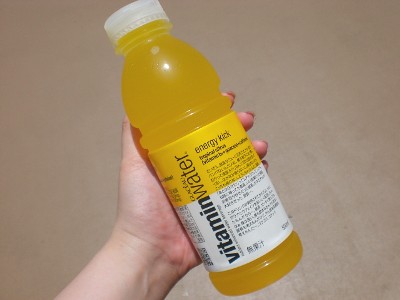In this photograph, a Caucasian hand, likely female due to the noticeable red nail polish and the hand's shape, is prominently holding a large bottle of Vitamin Water. The hand, with relatively long fingernails, is positioned palm open, showcasing all four fingers and part of the thumb as it grips the bottle. The bottle itself is notable for its size, appearing almost oversized in the grasp of the hand. 

The Vitamin Water inside the clear plastic bottle is bright yellow, and the bottle features a yellow and white label. Despite the small and somewhat blurry text, the label is partially readable and includes the product name, "Vitamin Water: Energy Kick." Below this, fainter text indicates nutritional information written in an Asian kanji script, suggesting that this product is marketed in a non-English-speaking country. The bottle is sealed with a clear plastic screw cap.

Set against a plain beige background, the image focuses entirely on the left hand holding this 500ml bottle, whether for an Instagram post, personal display, or possibly an advertisement.